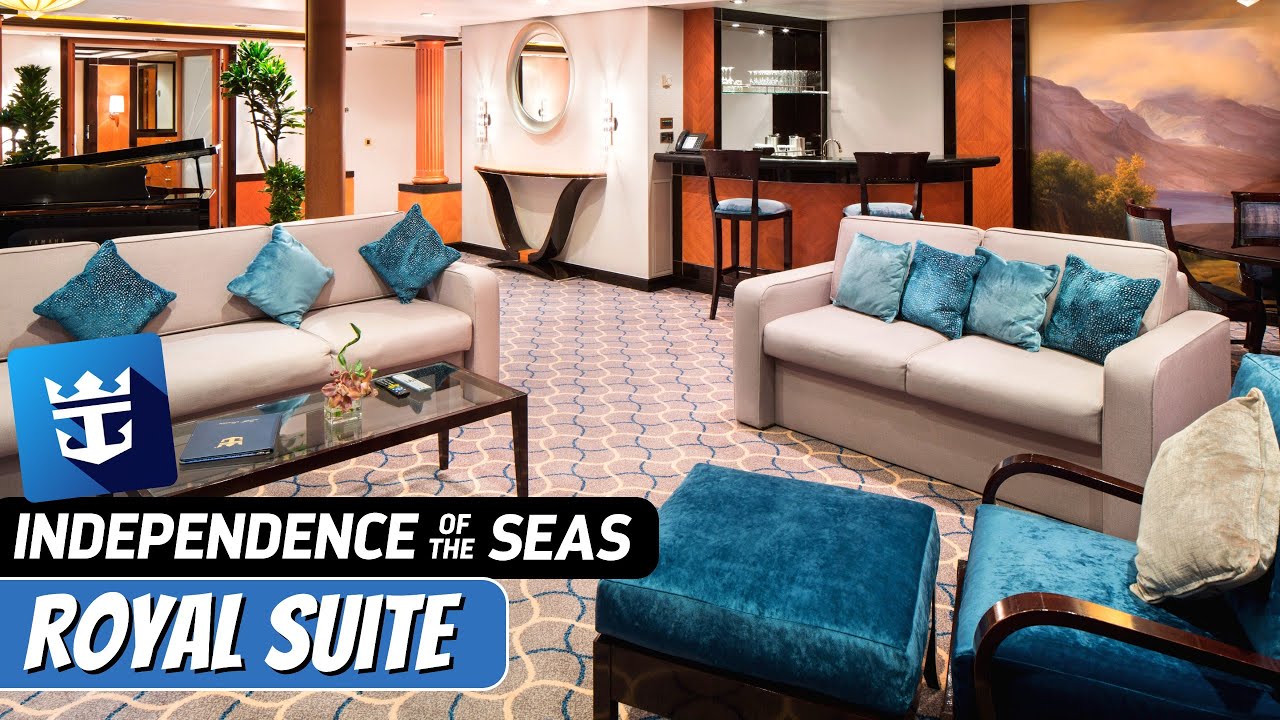This color photograph, intended for an advertisement, showcases a grand and well-lit living room environment in the "Independence of the Seas Royal Suite." The expansive room, which features gray carpeting with white and blue lines, is furnished with a carefully arranged furniture set including two gray-beige couches adorned with a total of seven blue pillows, a blue chair, and a blue ottoman. A glass coffee table with wooden legs, topped with papers and a flower, is positioned centrally. 

In the background, there's a stylish bar area with two gray and wood bar stools against a brown wood wall panel. A black grand piano sits prominently in the room. The wall includes a circular mirror next to two mounted lights. Additionally, there is a white table with a black base, a brown table, and a beige and blue rug that adds to the room's cohesive design.

A large wall mural and a glimpse of a dining room table can be seen, further emphasizing the room’s spaciousness. The advertisement text, which reads "Independence of the Seas Royal Suite" in bold white letters, is located in the lower left corner against a black and blue bar. This text is accompanied by a white anchor icon, enhancing the luxurious and nautical theme of the room. Plants strategically placed within the room add a touch of natural elegance to the sophisticated and clean interior.